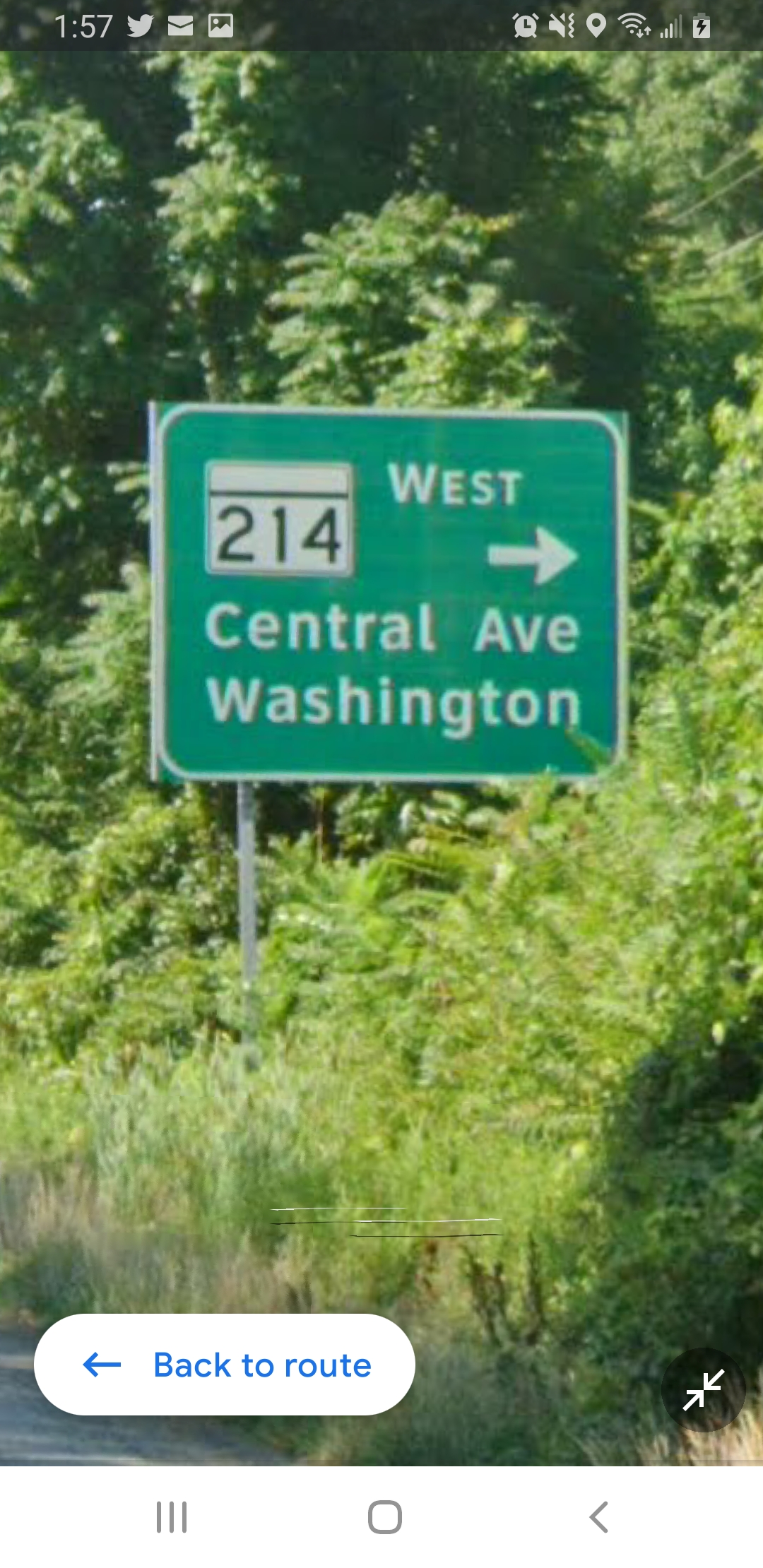This image is a screenshot of a smartphone display. At the top of the screen, the time is displayed as 1:57, accompanied by various icons and symbols typical of a smartphone interface. The main portion of the image showcases a photograph dominated by lush greenery. Amidst this green foliage, a street sign stands prominently. 

The street sign is mounted on gray metal poles. The sign itself is green with white text. It reads "West 214 Central Ave Washington," and features a white arrow pointing to the right side of the image. The number "214" is enclosed in a white box with black numerals and an additional black line above it, set against the green backdrop.

At the bottom of the screen, there is a white button labeled "Back to Route," accompanied by an arrow symbol, indicating a navigational option for the user.